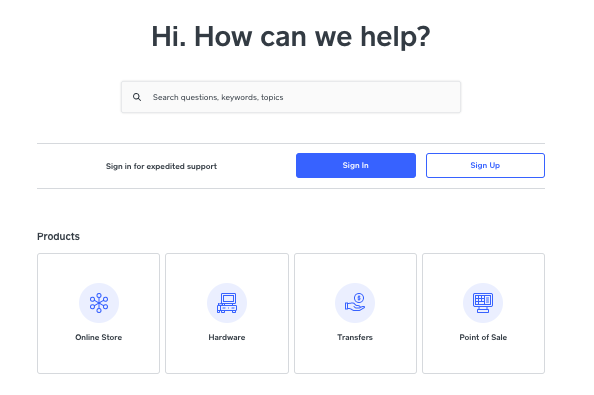The image is a screenshot of a website help page. At the top of the page, there is a prominent heading that reads, "Hi, how can we help?" Directly beneath this heading is a large search bar adorned with a magnifying glass icon. Inside the search bar, placeholder text prompts users to "search questions, keywords, topics."

Below the search bar, there is a smaller section dedicated to expedited support. This section contains two buttons: one blue button labeled "Sign In" for users who already have an account, and a white button with a blue border labeled "Sign Up," intended for new users to create an account.

Further down, the page features the heading "Products" followed by four outlined squares, each containing an icon and a descriptive word. The first square has a gray circle with an icon resembling a spoke wheel and is labeled "Online Store." The second square also has a gray circle, this time with an icon depicting computer hardware, labeled "Hardware." The third square shows a gray circle with an icon of a hand holding a small circle with a dollar sign, labeled "Transfers." The final square features a gray circle with an icon that looks like a computer functioning as a cash register, labeled "Point of Sale."